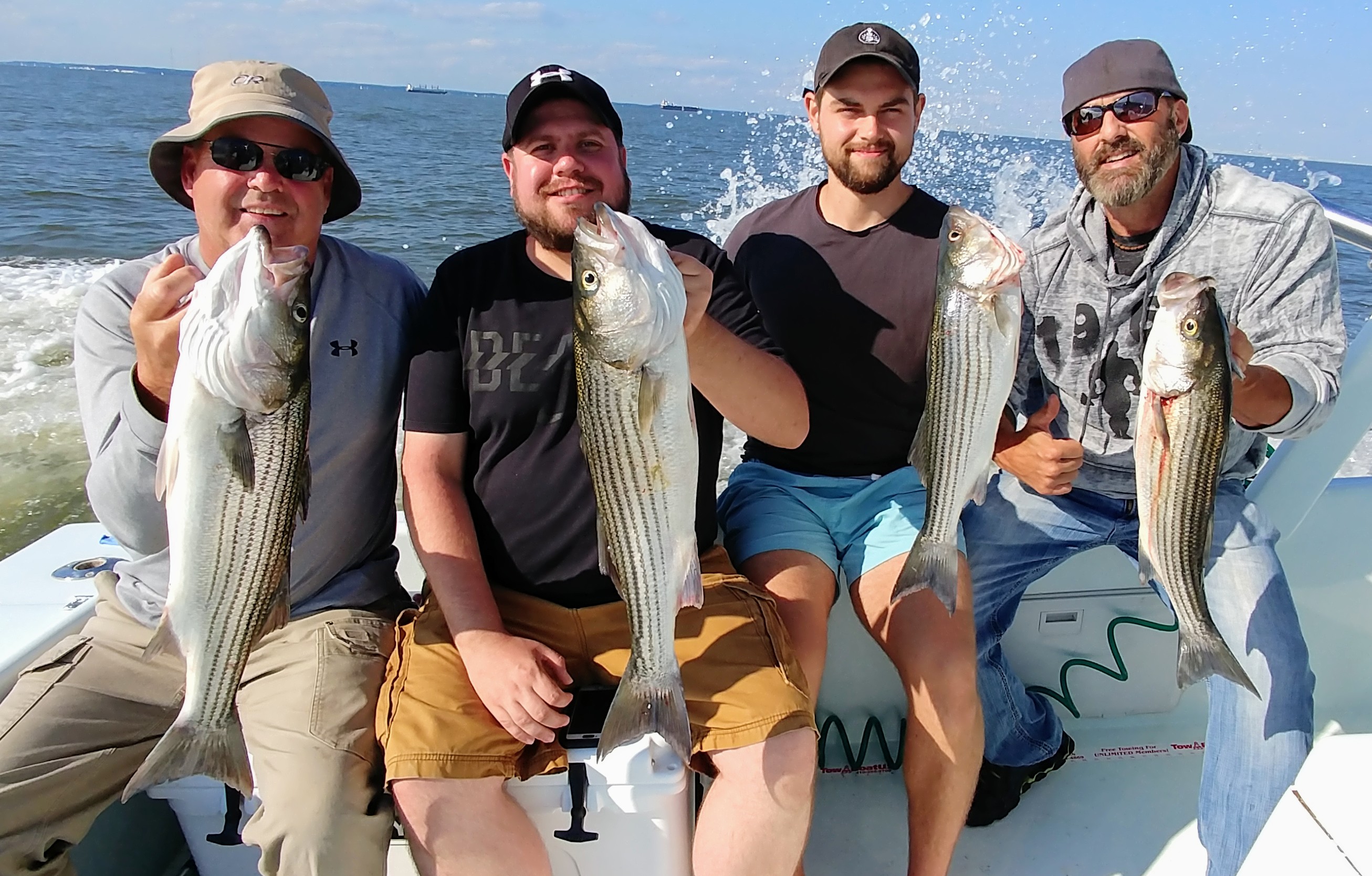The image features four fishermen seated on a boat in the middle of the ocean, proudly displaying their catches. The boat is moving, as evident from the splashing water and bubbles in the background stirred up by the propeller. All four men are holding up fish of the same species, characterized by grayish bodies with greenish-brown stripes running along their sides. They vary in size, with the larger fish held by the two men on the left.

The man on the far left is in his 40s, wearing a tan bucket hat, light blue zipped jacket, and tan pants. The second man, appearing to be in his 30s, sports a ball cap, blue t-shirt, and dark tan shorts. The third man, also in his 30s, wears a ball cap, blue t-shirt, and light blue shorts. The man on the far right, in his 40s, wears a beanie cap, long-sleeved hoodie, and blue pants. Both the first and last men wear sunglasses.

The sunny weather highlights their cheerful expressions as they showcase their catch, indicating a successful deep-sea fishing trip.